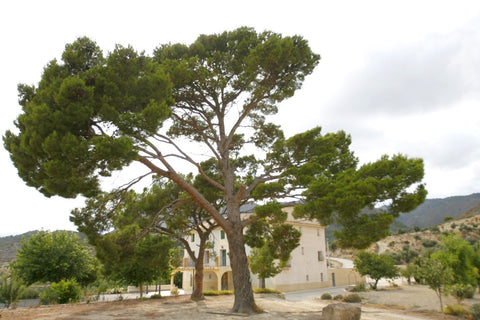This photograph captures a serene natural landscape with a central focus on a towering, verdant tree with dense foliage towards its ends and a sparse middle. This enormous tree partially obscures a grand, white three-story house or building, potentially used for residential purposes or special events, featuring a small balcony and a yellow porch. The house is set against a backdrop of distant mountain ranges with a mix of bare, rocky slopes and occasional greenery, lending a natural gradient of earthy tones to the scene. The foreground is dominated by a dirt and stone ground interspersed with smaller trees and bushes. On the far left and right of the image, there are additional small trees and bushes, framing the scene under a cloudy white sky. A driveway accented by rocks leads up to the house, hinting at the structured yet rustic charm of this picturesque location.